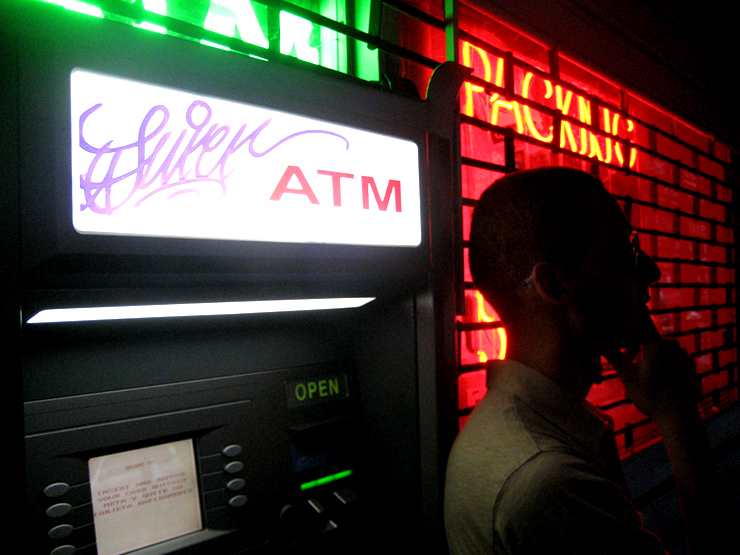In this nighttime image, a man stands silhouetted in front of an ATM machine. He is detailed with short-cropped hair, glasses, and a woven tan or gray collared shirt, holding his hand to his chin as if in thought or possibly on the phone. The ATM, situated on the left side of the image, is labeled with "ATM" in red on a white background, features a black body, a screen displaying "open" in green letters, and buttons for user input, beneath which is a green-lit card slot. The machine itself is marked with graffiti. Behind the man, the atmosphere is illuminated by red and green neon lights. The red neon sign spells out "packing," likely part of a storefront's signage. This storefront is secured by a closed metal gate, typical of urban environments like New York City. The scene's contrasting lights and shadows add a striking urban cityscape feel to the image.